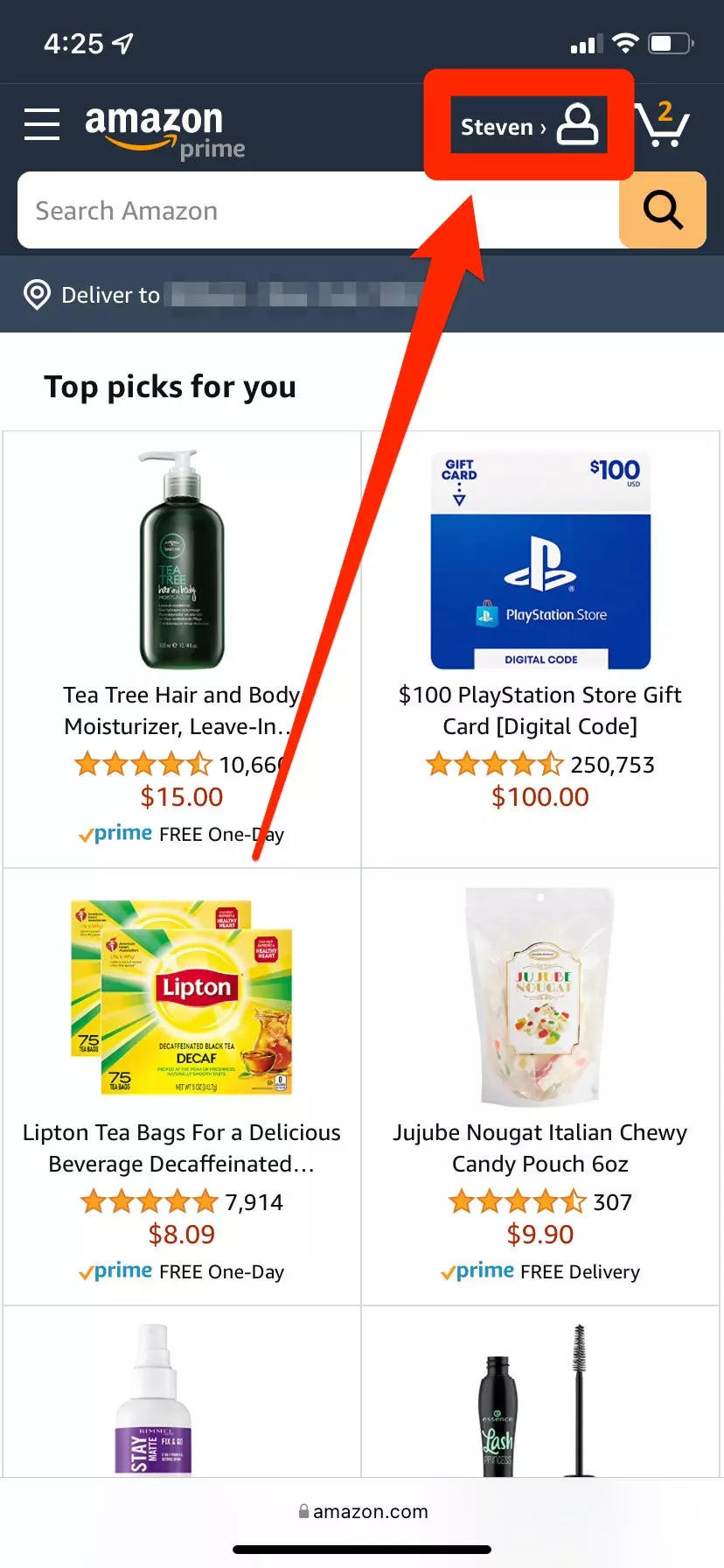In the image, there is a prominent black background at the top forming a large black box. In this section, the digital clock reads "4:25". Below the time display, there are three white lines followed by the word "Amazon," underlined with a red line, and "Prime" written in blue. To the right, the name "Steven" is featured alongside a small, head-and-shoulders icon, which is outlined in red. A bold red line surrounds this segment.

Adjacent to Steven's name, there's a small shopping basket icon with the number "2" in it, indicating items in the cart. Below this, there are various interactive elements including a search button and a "Deliver to" option.

The main content is titled "Top Picks for You," showcasing personalized product recommendations. The first recommended item is a "Tea Tree Hair and Body Moisturizer" priced at $15. Next is a "$100 PlayStation Store Gift Card" with a digital code, priced at $100. Following that, there's a pack of "Lipton Tea Bags," decaffeinated, priced at $8.09 with a "Prime Free One-Day" delivery option highlighted.

A conspicuous red arrow points upwards toward Steven's name, drawing attention. Lastly, there's an image of a pouch labeled "Jujube Nougat Italian Chewy Candy," 6 ounces, priced at $9.90. The image also displays the top portion of two other products, and at the bottom, "Amazon.com" is written next to a lock icon, followed by a black line underneath.